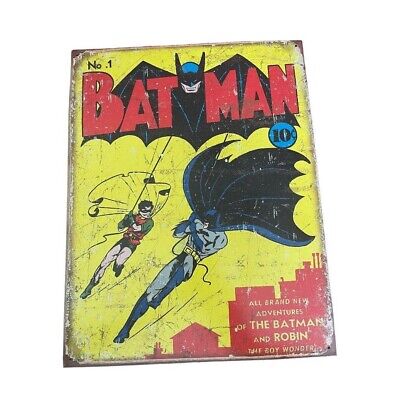Image Caption: This image showcases the highly coveted first issue of the Batman comic book series, a vintage treasure likely worth a significant amount of money. The cover proudly announces "All Brand New Adventures of the Batman and Robin, the Boy Wonder," possibly marking Robin's debut as the Boy Wonder. Priced at ten cents, this antique comic features Batman and Robin dynamically swinging on a rope against a striking yellow background, with a red cityscape below. The title is prominently displayed at the bottom. The comic, probably from the late 1930s or 1940s, appears aged with frayed corners. The iconic Batman logo, depicting Batman spreading his wings, is emblazoned at the top.